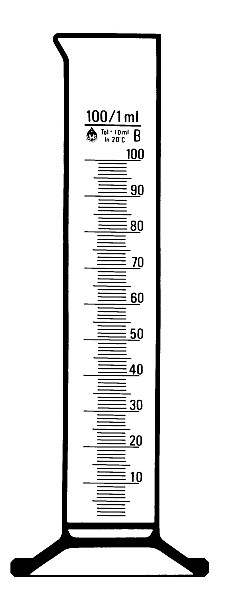This detailed drawing features a very tall and slender measuring vial, meticulously rendered in pencil with bold borders defining its edges. The unique illustration shows the vial equipped with two legs extending horizontally from both its lower corners. These legs are connected by a very thick black border, which itself supports another slightly thinner but still prominent black border above it.

Towards the upper part of the vial, measurement lines incrementally climb from 0 at the base to 100 at the top. Notably, the 0 line is left unlabeled. At the top, a clear marking reads "100 out of 1 mL," accompanied by a thick line just beneath it, followed by some smaller, finer text. Additionally, a note at the midway point indicates 20 degrees Celsius, or centigrade. Dominating the upper portion of the vial is a large "B" positioned above the "100" marking.

Finally, adding a touch of geometric interest, the left side of the vial's lid features a small triangle shape, completing the detailed and distinctive visual portrayal of this scientific instrument.